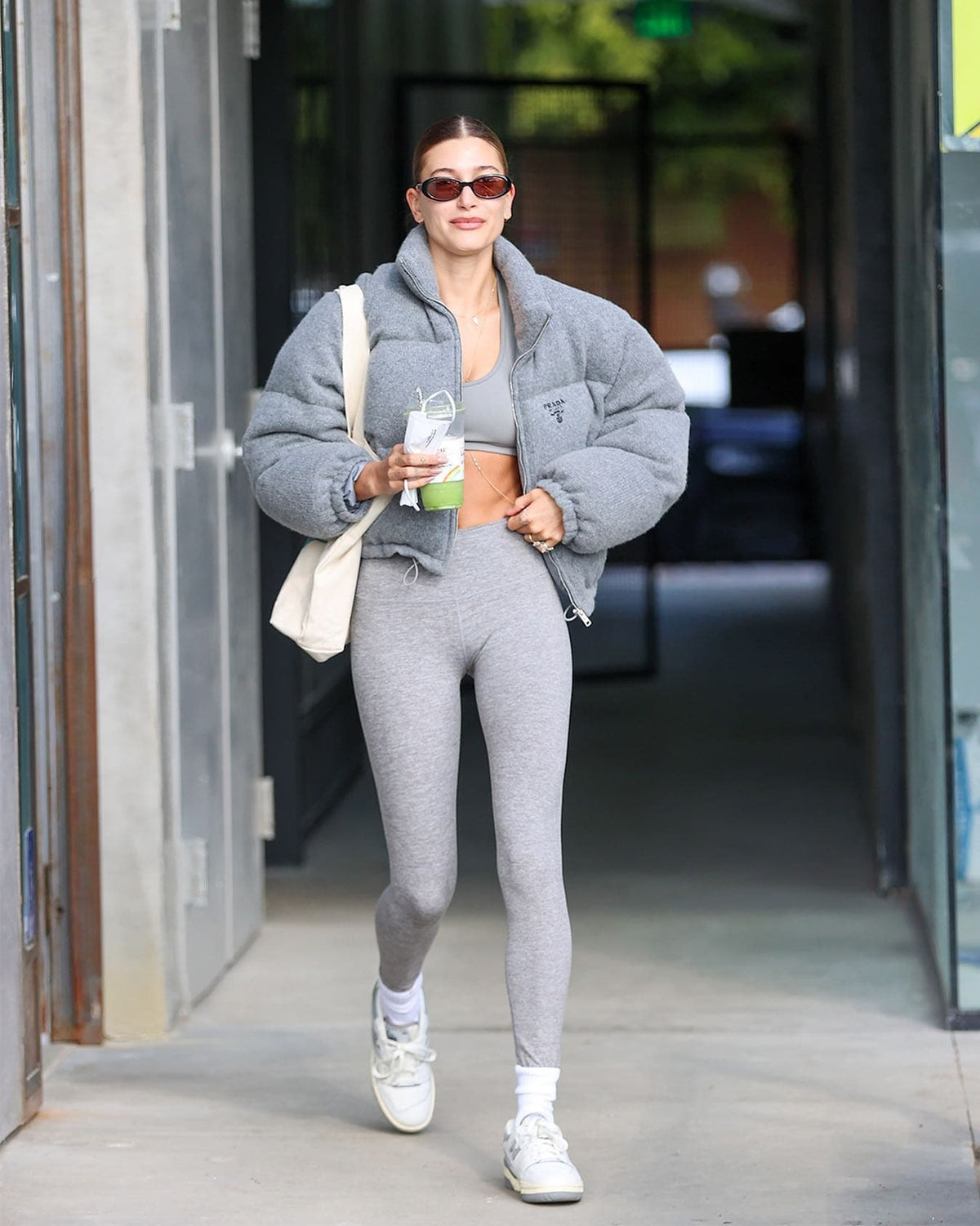This image captures a young woman in her mid-30s to early 40s, walking out of an apartment building on a sunny day that appears to be warm despite her large gray puffy winter jacket. She's wearing a gray sports bra under the jacket and gray form-fitting spandex pants that stretch down to white socks and matching white sneakers. On her head, she has dark amber-colored sunglasses with black frames, and her brown hair is parted in the middle and pulled back into a tight bun. The woman is of European descent and has rings on her left pinky and ring fingers. She carries a white tote bag over her right shoulder and a clear cup with what looks like a healthy green drink, possibly matcha or a smoothie, in her hand. She appears to be coming from a workout class, maybe yoga or Pilates, and is walking on a concrete surface with a noticeable smile on her face.